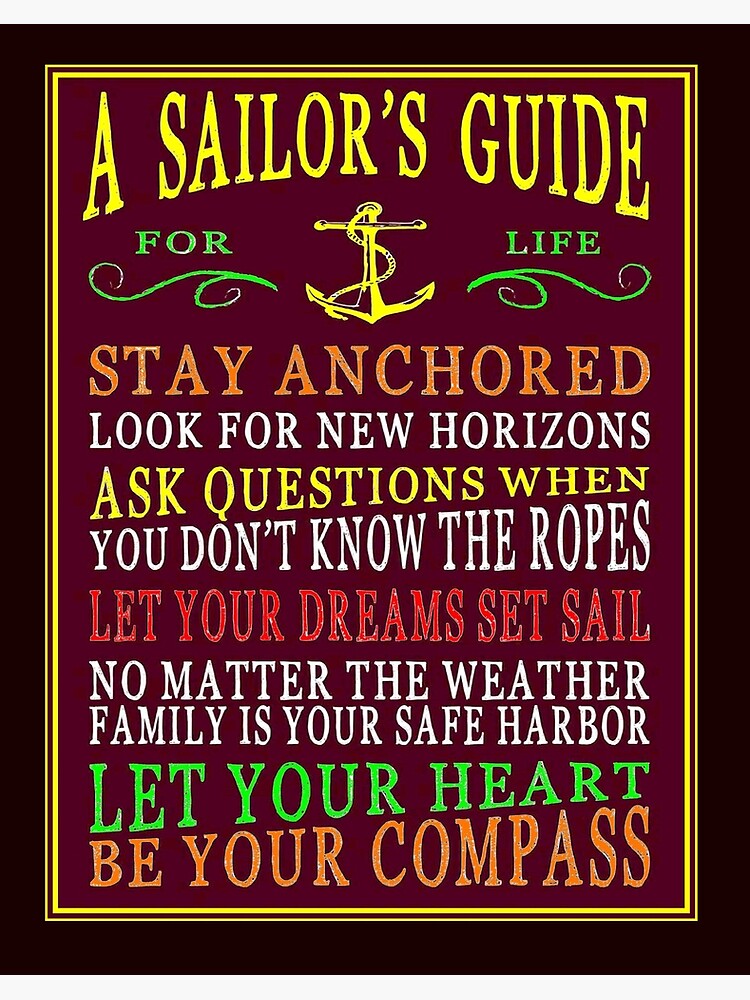This image depicts a decorative wall sign framed with a black border, followed by a thin yellow border, encapsulating a deep maroon background. At the top, in bright yellow all-caps text, it reads "A Sailor's Guide." Directly below this is the phrase "for life" with squiggly lines underneath, also in yellow, accompanied by a central emblem of a yellow anchor entwined with a rope. 

The sign continues with motivational phrases in varying colors: "Stay anchored" in orange, "Look for new horizons" in white, "Ask questions when you don't know the ropes" in yellow and white, "Let your dream set sail" in red, "No matter the weather, family is your safe harbor" in white, followed by "Let your heart" in green, and "be your compass" in orange. This sign combines encouraging nautical-themed advice with a vibrant, multicolored typography, making it a striking piece for wall decoration.